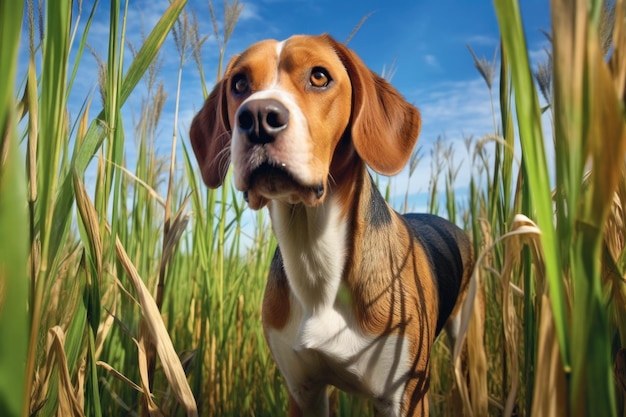A charming outdoor photo captures a beagle standing in a marshy or farm-like field with tall green and brown grass, possibly a wheat field. The beagle, with its typical coloring of brown, white, and black, has white markings around its nose, chest, and stomach, while the rest of its body displays a mix of brown with black on its back and neck. The dog, with expressive brown eyes and floppy ears, gazes intently into the distance, looking behind the viewer's left shoulder. The scene is bathed in daylight, with sunlight shining from the right, casting shadows on the right side of the dog. Above, the sky is a clear blue adorned with scattered light clouds, adding to the bucolic charm of this picturesque moment.